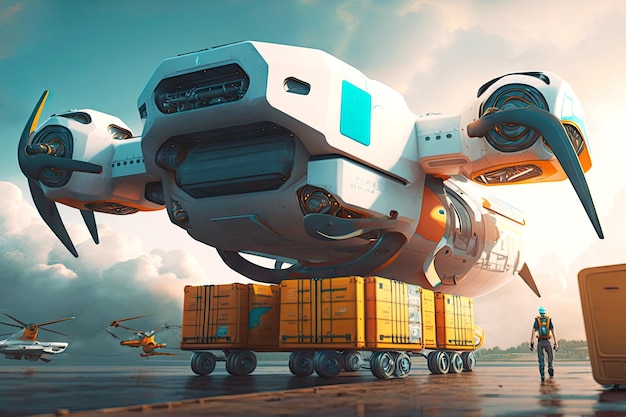This digitally rendered piece of art presents a futuristic and imaginative airfield scene. At the center, a series of yellowish-orange freight carts with at least five wheels each, some appearing sketched or incomplete, are seen traversing a shiny, wet surface. Resting atop these carts is a large, futuristic, white aircraft adorned with mismatched, curved propellers on either side. The aircraft appears to be hovering just above the freights or being transported by them. The left side of the sky shifts from a dark blue to a lighter hue towards the center and then transitions into pink and gray clouds on the right. In the bottom right corner, a man in safety gear, including a helmet and an orange vest, walks towards the viewer, suggesting his role at this airfield. Additional aircraft, small and slightly misshapen, hover close to the ground in the background, reinforcing the surreal quality of this scene.